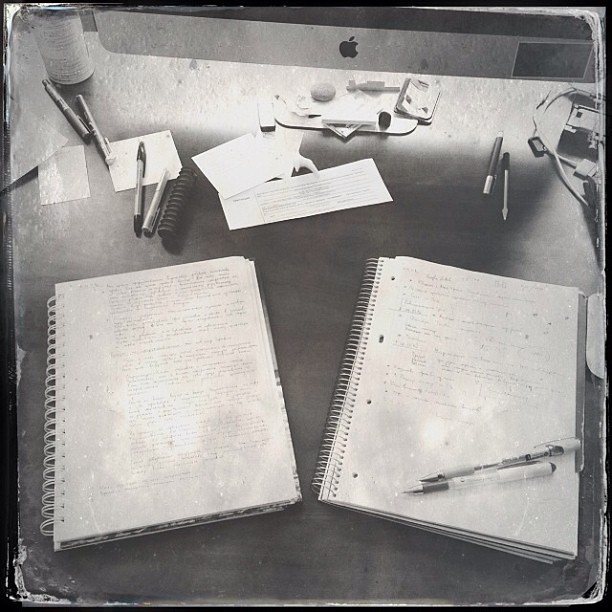This black-and-white photograph captures a detailed view of a professional desk setup. At the bottom, we see two spiral-bound notebooks laid open, one to the left with a thicker plastic spiral and the other to the right with a thinner metal spiral. Both notebooks are filled with handwritten notes, although the text is too blurry to read. The notebook on the right has two pens clipped open, ready for use resting on its pages. Moving upward, a collection of items scatters across the wooden table surface. Centered towards the top are Post-it notes and a variety of pens totaling at least six, along with folded papers and some electronic cords. In the top left corner, an unopened can sits on the table. The uppermost section of the image features the bottom part of a Mac desktop, identifiable by the Apple logo. The image, entirely monochromatic with shades of black, white, and gray, provides a comprehensive look at an organized yet busy workspace.